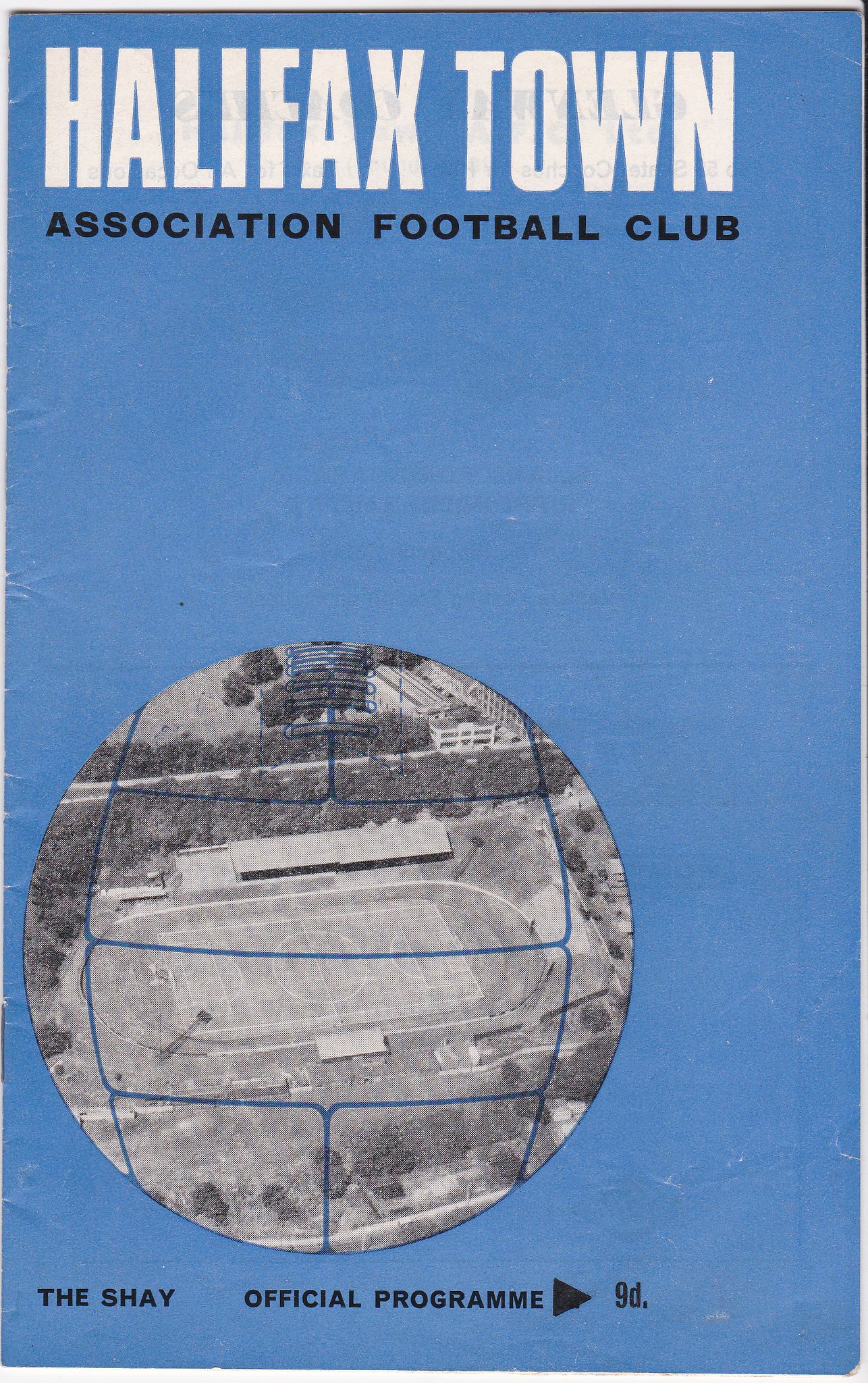The image is a single page from an old-fashioned football program for the Halifax Town Association Football Club. The background is predominantly blue, and at the very top left, bold white lettering reads "Halifax Town," followed by "Association Football Club" in black print just beneath it. Dominating the middle of the page is a circular black-and-white photograph depicting a bird's-eye view of a football field, surrounded by abundant greenery and some buildings in the distance. The circle with the football field image is designed to resemble a soccer ball, complete with laces at the top section. At the bottom left corner of the page, "The Shea" is printed, followed by "Official Program" to the right, accompanied by a black arrow pointing right and the characters "9D." The layout solely focuses on this single, regular-sized program page, highlighting its retro aesthetic and detailed imagery.